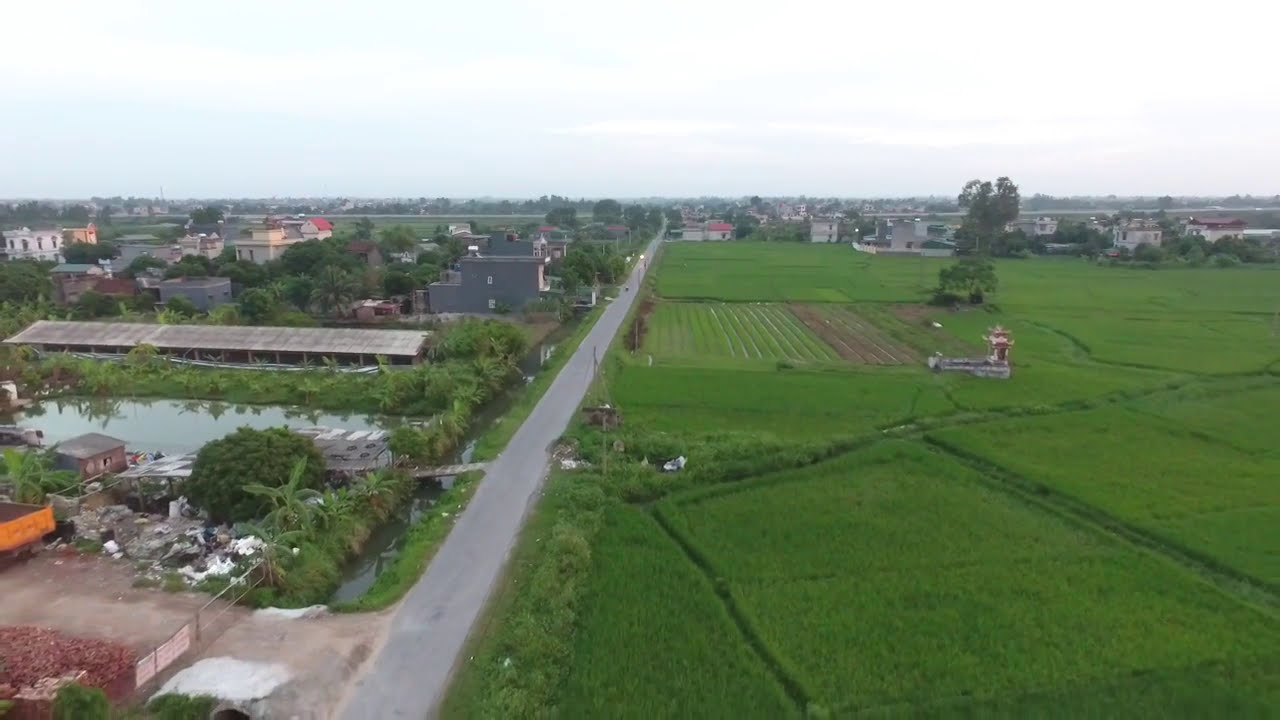The image captures a shallow aerial view of a flat farm landscape, elevated about 30 feet above the ground. The scene is divided by a narrow, gray, two-lane road that runs straight across the middle of the image, extending towards the white sky on the horizon, which appears about four-fifths of the way up the image.

On the right side of the road lies a vibrant, bright green field, sectioned off into large rectangles, indicative of farming activities. The field features distinctive rows suggestive of crops growing and a large tree standing prominently in the middle. Few trees are present, adding to the expansive and cultivated appearance of the farmland.

In contrast, the left side of the image portrays a more cluttered and run-down area. A small pond is visible near the center-left, adjacent to a parking lot that extends out of the frame. This area appears to be a construction site, littered with trash, debris, gray matter, and possibly bushes. A dump truck is notably parked in the lot, surrounded by scattered items and debris piles. Further in the background on the left, an assortment of buildings, possibly houses, stretches across the horizon.